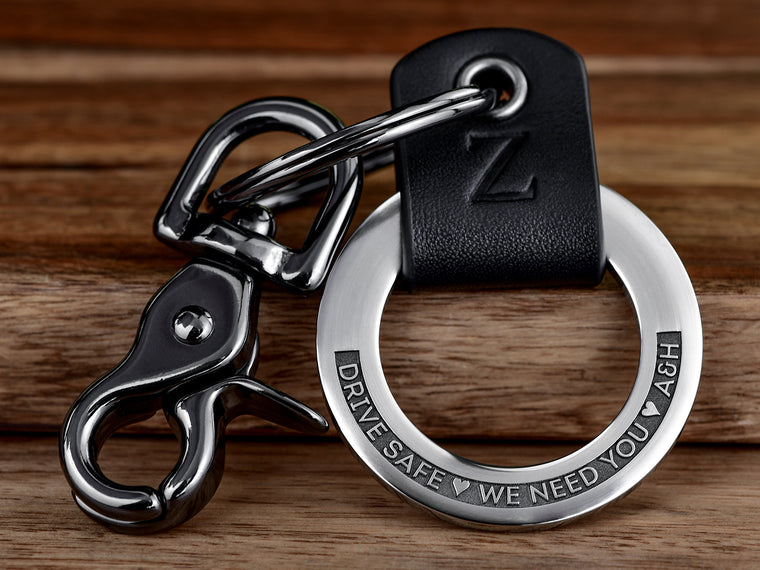This is a detailed close-up of a personalized keychain resting on a wooden table with horizontally aligned slats, possibly oak, transitioning into a slightly darker gradient towards the back. The keychain features a black leather strap wrapped around a sturdy silver ring. The strap has a leathery texture and connects to a clasp designed for attaching to a belt loop or key ring. 

The silver ring, thick and robust, showcases an intricately engraved message: "Drive safe ❤ We need you ❤ A&H." The engraving is highlighted by a black text box that frames the silver letters, making the inscription stand out clearly against the shiny metal backdrop. The heart symbols and letters add a heartfelt, personal touch to the keychain. This elegant and practical accessory combines silver and black elements, blending durability with a thoughtful message.